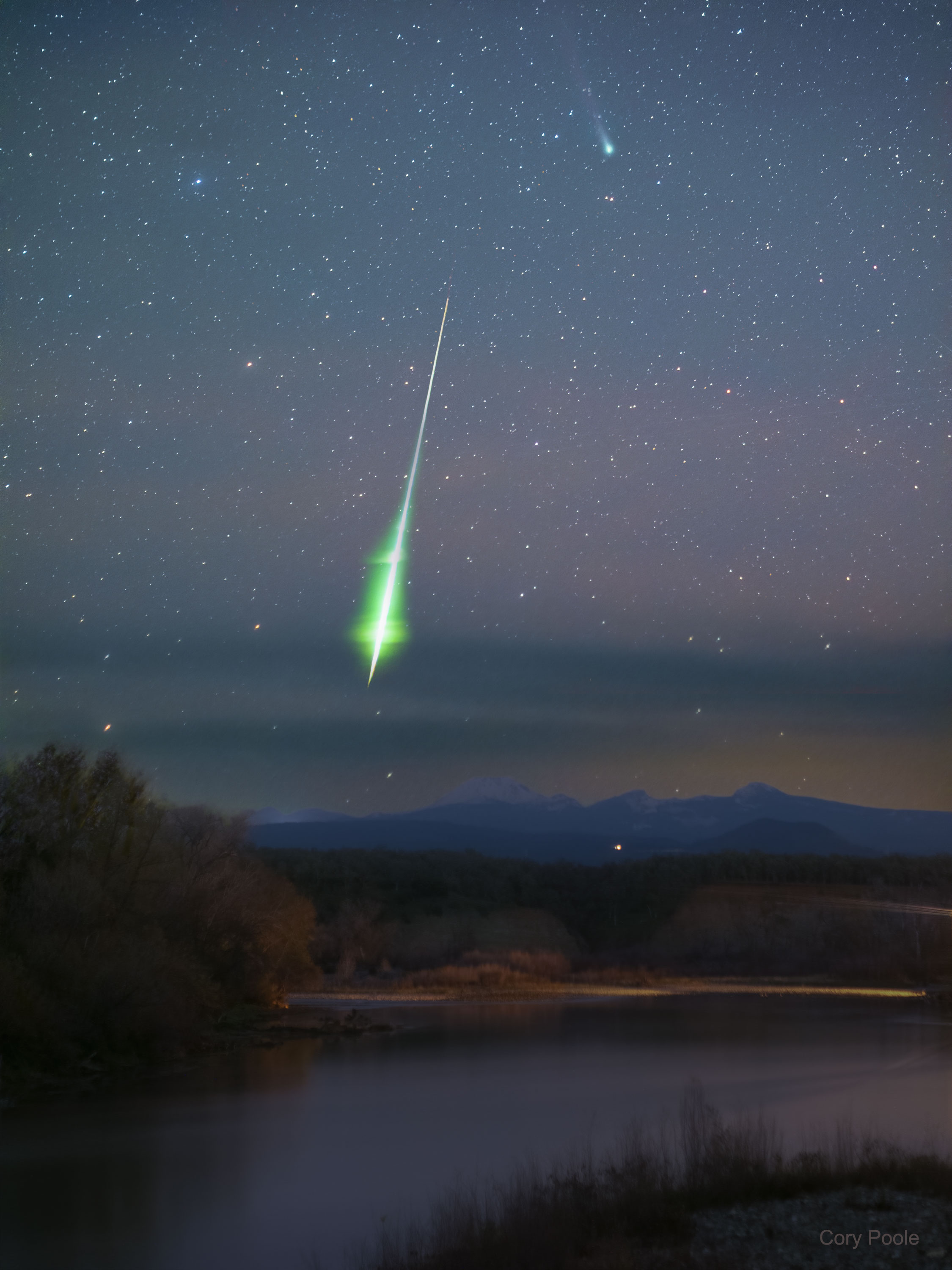The photograph captures a serene nighttime scene featuring a very still lake or pond, surrounded by a rocky foreground with patches of foliage and grass. In the bottom right corner of the image, the name "Corrie Poole" can be seen. The lake is bordered by some tall trees on the left side and a shoreline dotted with more trees. Behind this shoreline rises a series of hills and mountain ranges, whose snow-capped peaks are faintly visible despite the darkness. The night sky, the main focus of the image, is filled with dozens of bright white stars scattered across it. Two shooting stars are particularly notable: one, near the top of the picture, is slightly larger than the surrounding stars and has a faint, fuzzy tail, while the other streaks diagonally from the middle of the image towards the bottom left, casting a luminous green blur around its bright white core. There is a hint of light—possibly the first glow of dawn or another off-screen source—emanating from behind the mountains on the right side of the image, adding a subtle promise of daylight to come.